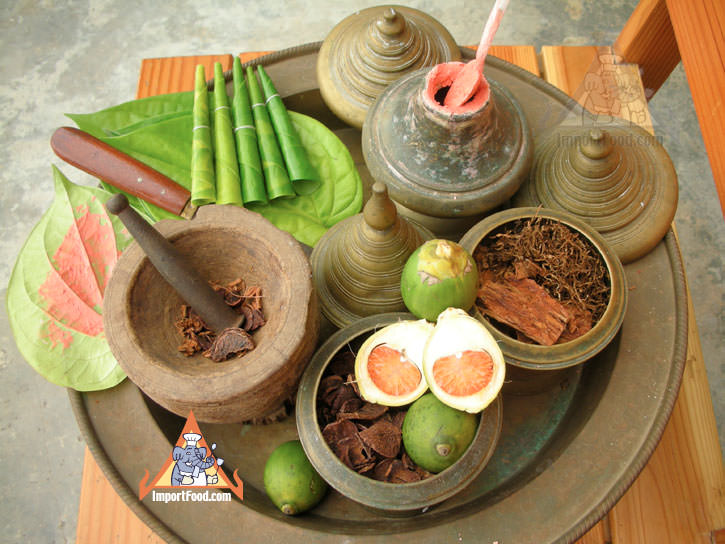The image showcases an aerial view of a rustic and visually intriguing assortment of food items on a wooden table, above a concrete floor. Centered on an antique-looking circular brass tray, the display includes an array of ceramic and clay-style dishes, each containing various spices, fruits, and leaves. Among them, a stone mortar and pestle with crushed herbs and spices stands out, positioned at the left. Adjacent containers, some with conical lids and others resembling jars, hold elements like cinnamon bark, an egg-like item with an orange center, green fruits, dried grass, and red paste with a spoon sticking out. In the background, meticulously rolled betel nut leaves sit atop a larger leaf, adding to the intricate arrangement. The scene is accentuated by a logo in the bottom left corner featuring a triangle with an elephant wearing a chef's hat, reading "importfood.com," which also appears as a translucent watermark in the upper right. The overall setup exudes a vintage, antique charm, emphasized by the grayish-green tint of the plates and the rustic, brass aesthetics of the containers.